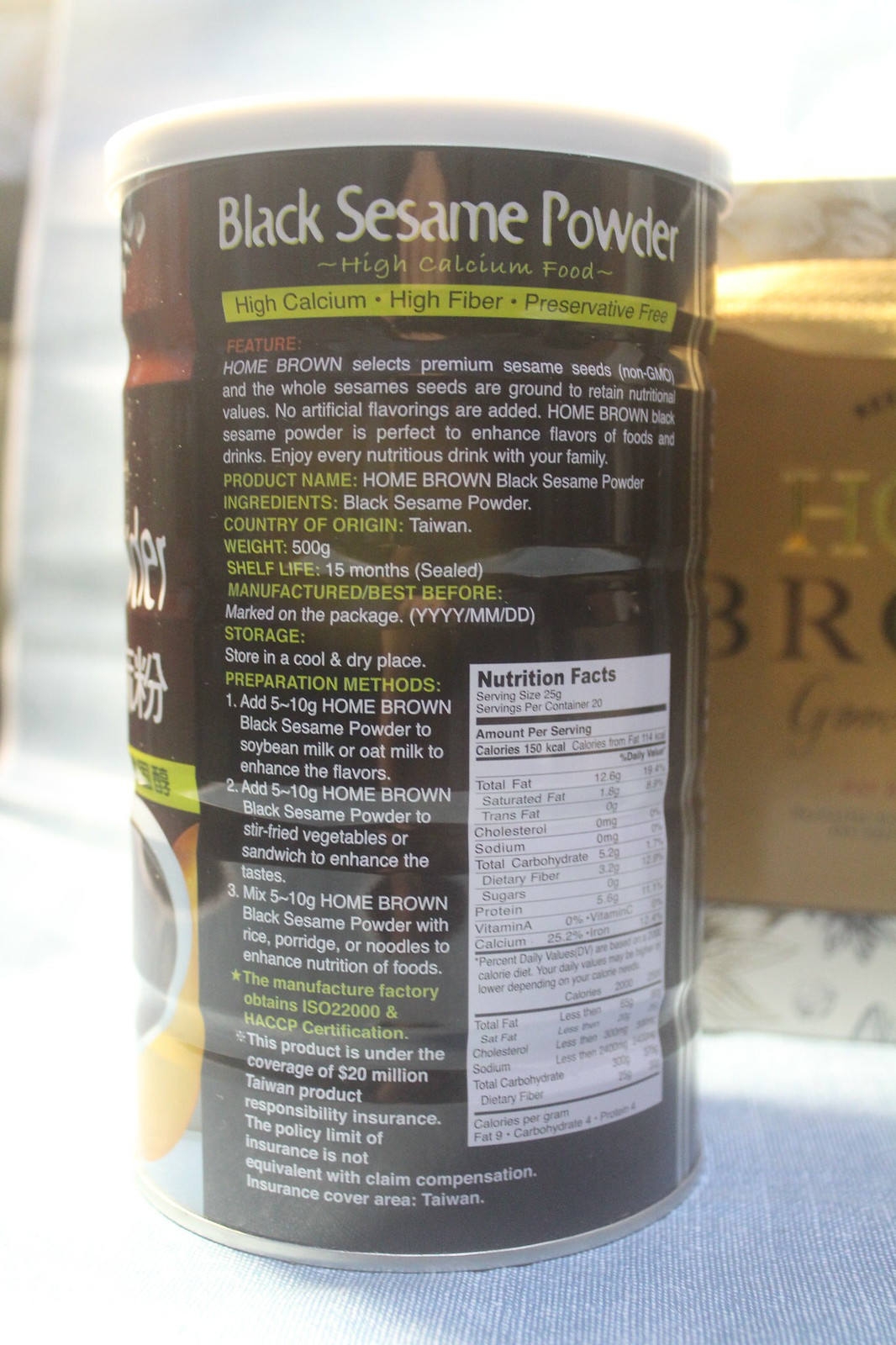The image depicts a cylindrical steel can of Black Sesame Powder from Home Brown, covered in a black label with white and bright yellow text. The can features a replaceable white plastic pop-on lid. We're viewing the back side of the label, where "Black Sesame Powder, High Calcium Food" is prominently displayed. Below it, a yellow bar states "High Calcium, High Fiber, Preservative Free." In the following sections, additional details are listed: 

- **Features**: Non-GMO, no artificial flavorings, made from premium sesame seeds ground to retain nutritional value. It is certified under ISO 2000 and HACCP standards.
- **Product Information**: The label contains information such as product name, ingredients (black sesame powder), country of origin (Taiwan), weight (500 grams), shelf life (15 months), storage instructions (store in a cool and dry place), and preparation methods. 
- **Preparation Methods**: Suggests adding 5 to 10 grams to soybean milk, oat milk, stir-fried vegetables, sandwiches, rice, porridge, or noodles to enhance flavors and nutrition.
- **Insurance Note**: The product is covered by a 20 million Taiwan product responsibility insurance policy, although the policy limit is not equivalent to claim compensation and only covers Taiwan.

A Nutrition Facts rectangle is also visible on the right side of the label.